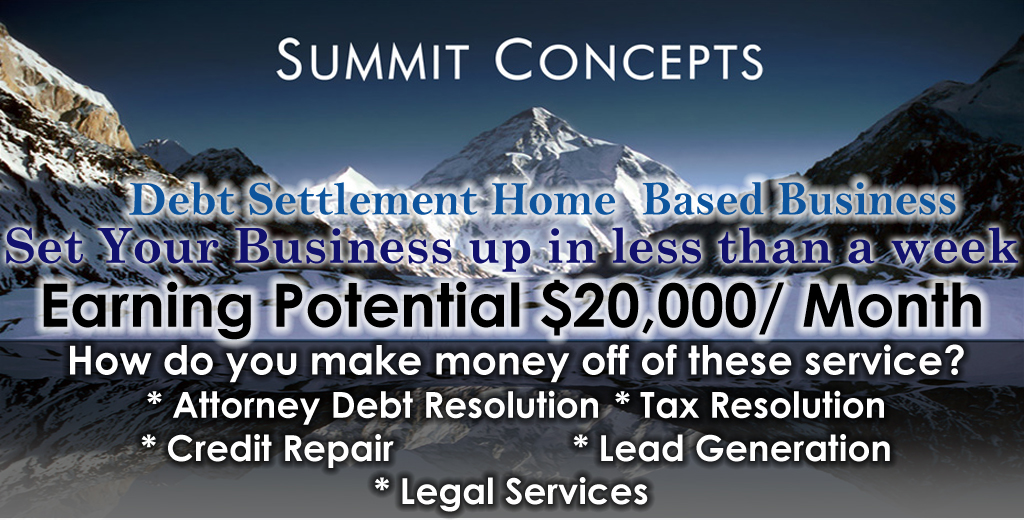The advertisement for Summit Concepts is set against a backdrop of rugged, rocky mountain peaks dusted with snow, under a dark blue sky suggesting early night. The business card has a horizontal and rectangular layout. Predominantly featuring text overlay, the card begins at the top center in white text with "Summit Concepts" standing out prominently. Below this, the text “Debt Settlement Home-Based Business” appears in blue, followed by “Set your business up in less than a week” in a darker blue. Further down, in bold black text on a white banner, it promises an “Earning potential $20,000/month”.

The caption continues in white text, asking "How do you make money off of these services?" and proceeds to enumerate the service offerings with asterisks: * Attorney Debt Resolution, * Tax Resolution, * Credit Repair, * Lead Generation, * Legal Services. The mountains’ varying textures and snow cover provide a striking visual context for the compelling text, effectively promoting the lucrative opportunities available with Summit Concepts.